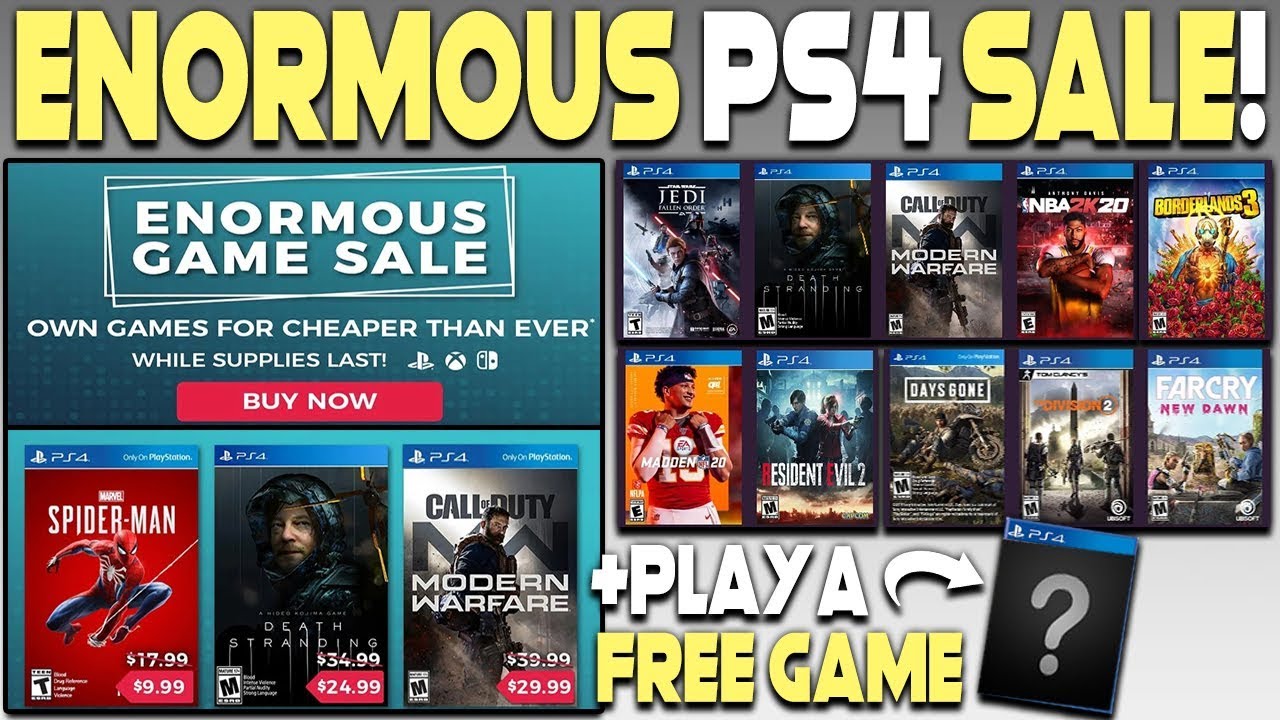The image depicts a vibrant advertisement for an enormous PS4 game sale. The headline features bold, eye-catching text: "Enormous" in yellow, "PS4" in white, and "Sale" with an exclamation point in yellow and white. This sale is substantial, offering a variety of discounted games. Highlights include the popular game "Spider-Man" available for just $9.99. The promotion suggests that there are additional games like NBA 2K and freebies available, enhancing the appeal. The placement of this ad is unspecified, potentially appearing in a newspaper or online.